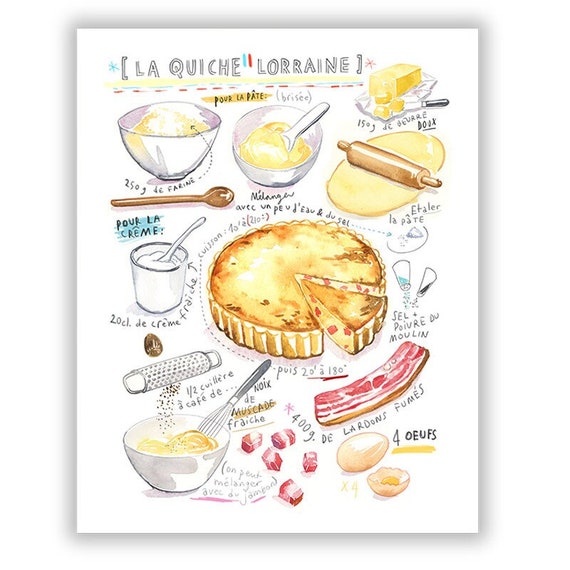This image is a detailed, illustrated recipe for "La Quiche Lorraine" set on a white background in portrait layout. In the upper left-hand corner, black text reads "La Quiche Lorraine," introducing the dish. The illustration uses vibrant colors including white, yellow, red, black, and blue. The sequence begins with a bowl in the top left containing a substance, potentially flour or cheese, and another bowl in the center holding a spoon. Adjacent to these is an image of butter being cut by a knife, followed by a wooden rolling pin flattening dough beneath it.

Next, there is a wooden spoon and a cup labeled "pour la creme." The upper right side displays the finished quiche with a slice missing. Below, there are images of salt and pepper shakers, indicating seasoning. In the middle section, a grater drops small black specks into a bowl being whisked, hinting at grated nutmeg. Beside this, there are small, cut-up red pieces of meat identified as bacon, along with a larger piece of bacon. In the bottom right, several eggs are illustrated.

The detailed visual steps show how to prepare the quiche, from mixing the initial ingredients, rolling out the dough, adding cream, grating nutmeg, cubing bacon, incorporating eggs, seasoning, and finally displaying the baked quiche in its completed form.